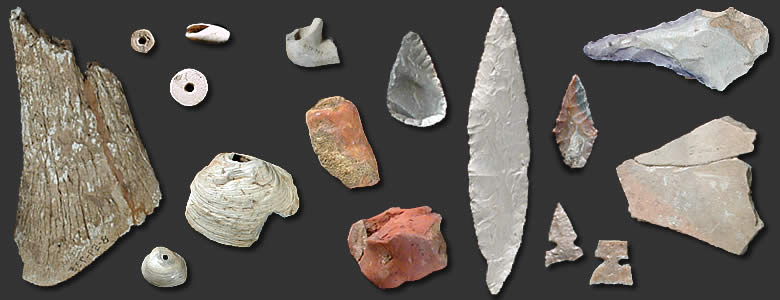The image portrays an assortment of found objects, likely from an archaeological dig, meticulously displayed against a black background. The collection includes an array of artifacts: on the left side, there is a piece of bone, various shell fragments, possibly oysters, and stones in shades of red and brown. Among these, some stones appear to be intricately carved into arrowheads, with two smaller ones flanking a longer piece that has arrowheads on both ends. Each smaller arrowhead has a pointed end and a blended end. Below these, two additional examples of carved weaponry are visible. On the right, two stones resemble those used to create tools. The collection also features what might be a piece of petrified wood and several rocks fashioned into pointed shapes, likely spears or cutting tools. Additionally, there are uniquely shaped stones, including cream, brown, and salmon-colored pieces, and two circular stones with distinct holes punched through them, indicating potential use as ancient jewelry or tools. The objects, seemingly primitive and possibly buried for a long time, showcase a glimpse into the past, documenting the types of artifacts unearthed in a specific region.